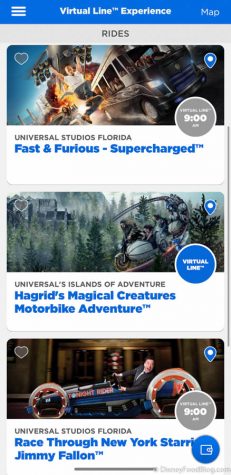This image is a mobile screenshot displaying an interface for managing virtual lines at a theme park. The mobile browsing environment and operating system are not visible in the screenshot. The top-left corner features a hamburger icon, symbolized by three vertical lines, which typically opens a menu of options. This icon is set against a medium blue background with the text "Virtual Line™ Experience" in bold white font. On the top-right, the word "Map" is also displayed in white text.

Directly below this header, the word "RIDE" is prominently featured in uppercase letters in a grayish-black font, denoting a section title. Beneath it are various ride options, each with a corresponding heart icon for favoriting and a map pin icon to indicate their location.

The first ride listed is "Universal Studios Florida - Fast and Furious Supercharged™." "Fast and Furious Supercharged" is highlighted in blue text with a trademark symbol (™), while "Universal Studios Florida" is in black uppercase text. There is an additional note mentioning a virtual line time of 9 a.m.

The next ride option is "Universal's Islands of Adventure - Hagrid's Magical Creatures Motorbike Adventure," which also features a virtual line system.

Following that is "Universal Studios Florida - Race Through New York Starring Jimmy Fallon™." Similar to the first ride, the name "Race Through New York Starring Jimmy Fallon" is in blue text with a trademark symbol (™), and "Universal Studios Florida" is in black uppercase text. A virtual line time of either 9 a.m. or p.m. is also mentioned.

In the bottom right corner of the screen, there is an icon that appears to represent either a notebook or a wallet, though its function is not entirely clear.

Overall, this image showcases various rides within a theme park that offer a virtual line system, seemingly designed to reduce the need to wait in physical lines.